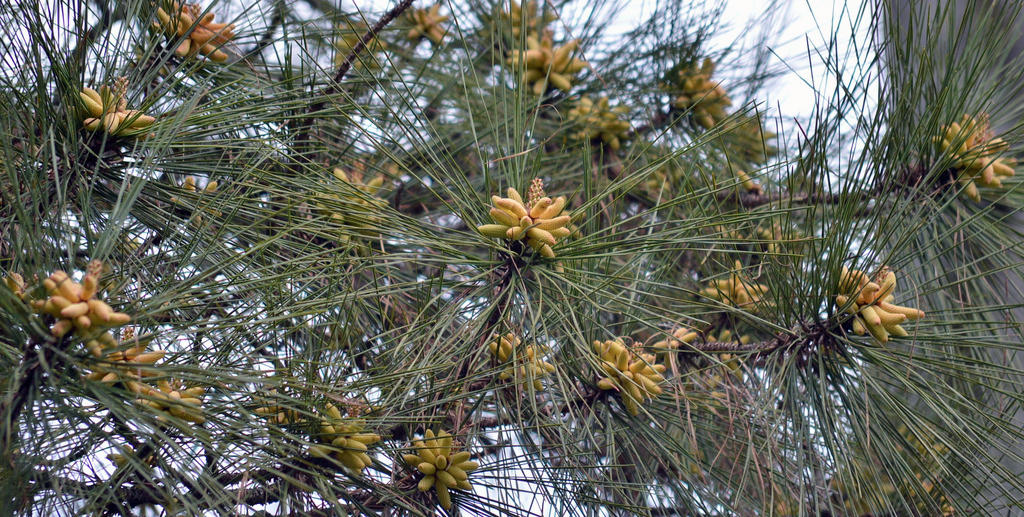This close-up photograph captures the intricate details of what appears to be a tropical or evergreen tree, possibly related to a pine tree, though its exact species is unclear. The camera is angled upward from the ground, focusing on the long, thin, pine needle-like leaves extending from dark brown branches. At the center of these branches are clusters of yellowish-orange fruits or underdeveloped pine cones, approximately an inch long and resembling miniature fingers. These clusters are scattered among the green needles, adding a burst of color to the composition. The branches span across the frame, with numerous small offshoots densely packed with needles and fruits, creating a rich tapestry of foliage. In the background, a bluish-white sky filters through, illuminating the scene with a soft, natural light. On the right side, a faint image of what might be a tree trunk suggests the presence of a larger tree just beyond the frame. The overall impression is one of vibrant natural beauty, showcasing the detailed textures and colors of this unidentified tree species.